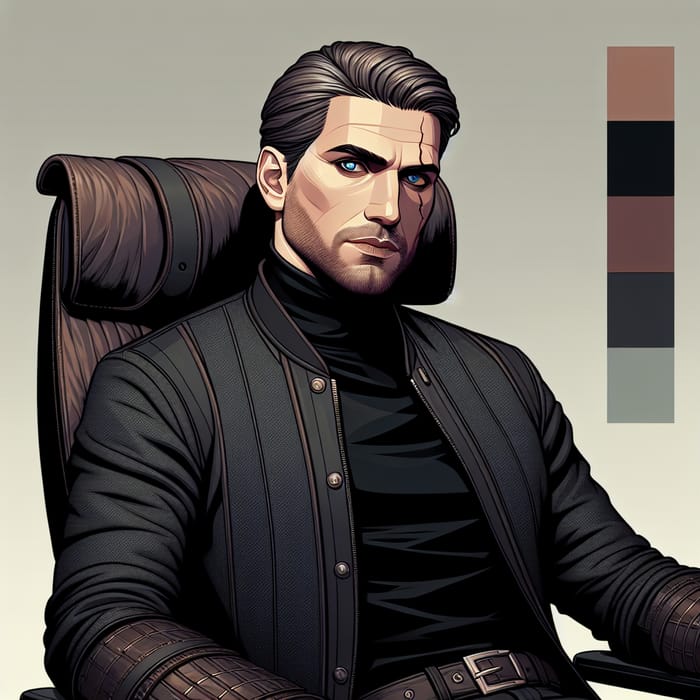This detailed image portrays a computer-animated, cartoon-like painting of a man with striking features. The man, who evokes a resemblance to a well-known actor, sits facing forward in a brown-colored leather chair. His dark brown hair and thick eyebrows frame his piercing blue eyes, which almost seem to glow. A notable scar runs vertically from his forehead down past his left eye, adding to his striking appearance. He has a chiseled nose, a subtly cleft chin, and a faint goatee. The man is dressed in a black turtleneck paired with a black leather jacket and a black belt featuring a silver buckle. His arms rest on the armrests of the chair. The background is predominantly gray, transitioning from a lighter to a darker shade, and on the right side of the image, there is a rectangular color swatch. The swatch includes blocks of various colors: light brown, black, dark brown, dark gray-black, and grayish-green, though it appears incomplete, missing some of the lighter background and skin tone shades.